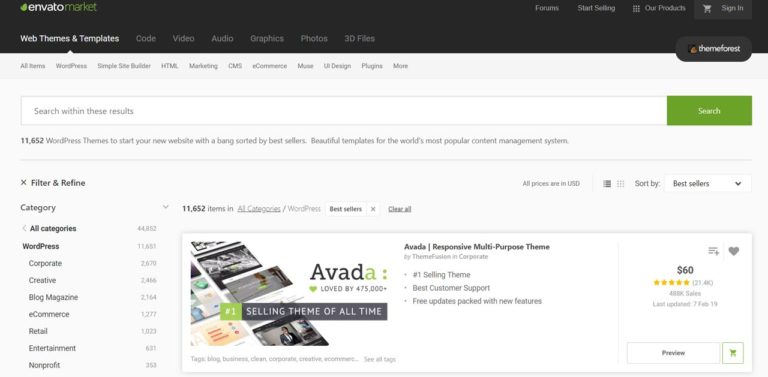The image depicts the homepage of the Envato Market website. In the upper right-hand corner, the words "Envato Market" are displayed, with "Envato" in white and "Market" in green. To the left of the word "Envato," there is a green icon. The image has various text across the top, including options such as "Start," "Start Something," which are faint but readable, as well as "Forum," "Start Selling," "Our Products," "Sign In," and a shopping cart icon.

Beneath this, the logo "ThemeForest" is prominently featured. Below the logo, there are several categories listed, although they are very light and unreadable. A search bar is present with the word "Search" in green next to it. Directly below, there's a filter option labeled "Filter to Refine," with various categories such as WordPress, Corporate, Creative, Blog Magazine, eCommerce, Retail, Entertainment, and Non-Profit.

In the main body of the image, there is a banner for "Avada," boasting as the "Most Loved Theme of All Time" with over 475,000 sales. It shows an image of business cards laid out on a surface and promotes the "Avada Responsive Multi-Purpose Theme." It highlights its features as the "#1 Selling Theme," "Best Customer Support," and promises "Free Updates Packed with New Features." On the right side, the theme is priced at $60 and has a five-star rating in yellow.